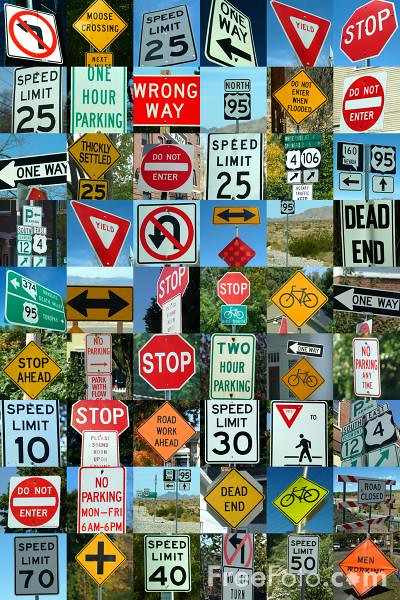This image is a detailed collage of 54 diverse road signs, each displayed in small, uniform, rectangular photographs arranged in a 6x9 grid. The majority of the signs are red stop signs, depicted from various angles, including straight-on and diagonal views. Among the plethora of signs, one can spot no left turn and no u-turn signs, numerous speed limit signs ranging from 10 to 70, and moose crossing signs. Other notable inclusions are diamond-shaped warning signs such as dead end, stop ahead, and those with a bicycle symbol, as well as rectangular signs like road closed and do not enter when flooded. Each photograph features different backgrounds from blue skies with tree lines to snippets of roads. At the bottom, a watermark indicating "freephoto.com" hints at the compilation's origin, potentially serving as an advertisement showcasing the variety of road sign images available from this source.